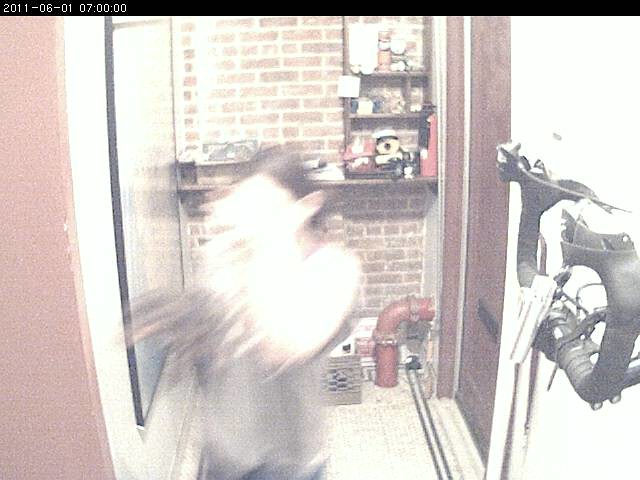In the photograph, a person in motion appears blurred, contrasting with the sharp details of the surrounding setting. The scene unfolds in a hallway featuring a brick back wall, against which a built-in shelf is positioned. A prominent red metal pipe emerges from the floor, bends, and enters the wall beneath the shelf. A can of Raid sits atop the shelf. To the right, a dark red door with a mail slot at the bottom stands out, along with its threshold. On the left wall, a large picture in a black frame draws attention. The lady in the image has her hair parted in the middle, and behind her, in front of the brick wall on the floor, rests a brown milk crate.